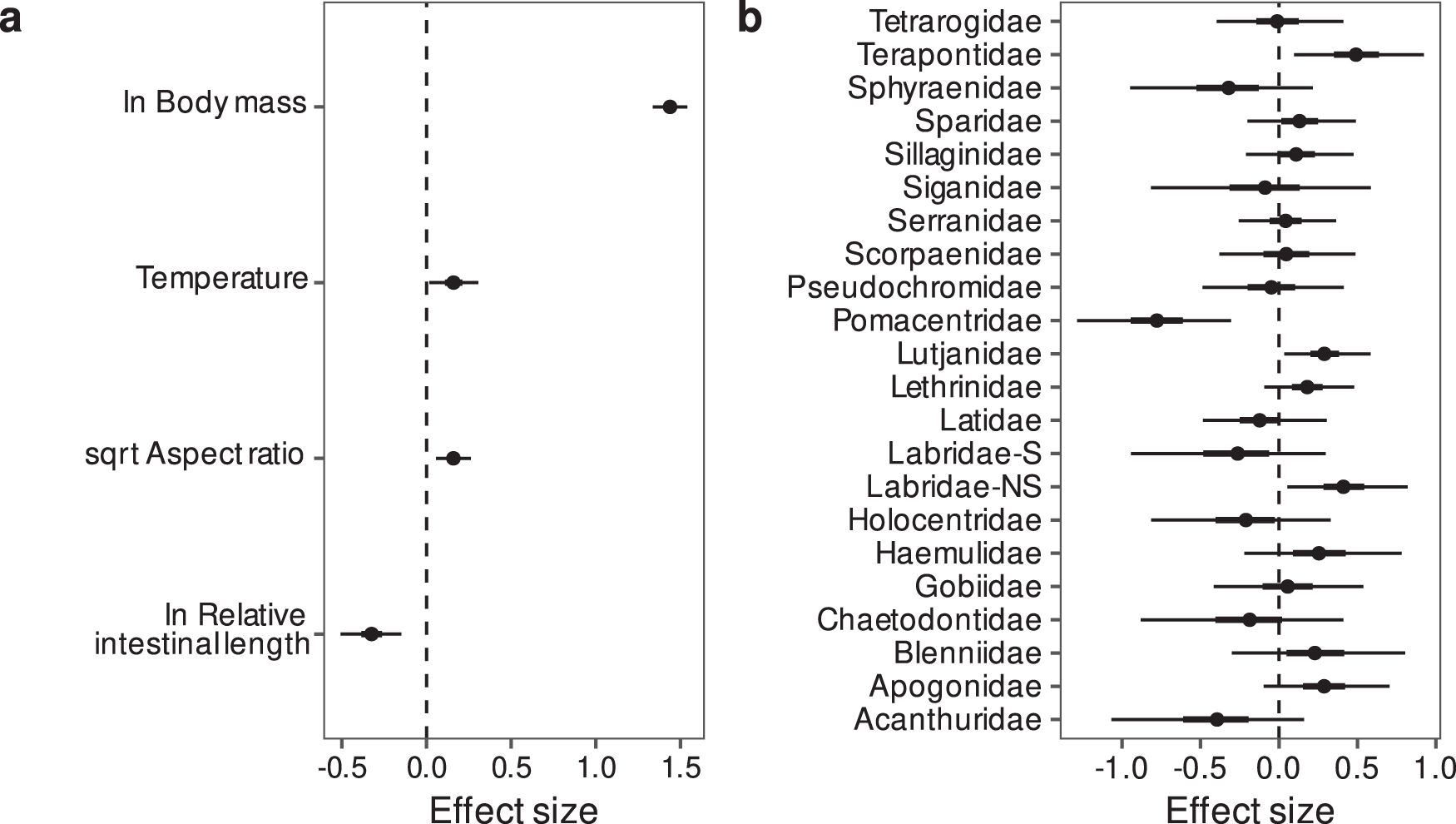The image is a side-by-side scientific diagram with two sections labeled A and B, each illustrating the effect size on a horizontal axis. The effect size in both sections is measured in 0.5 increments. Side A features a long rectangular box with a dashed line down the left side. It lists four categories on the vertical axis: body mass, temperature, square root aspect ratio, and relative intestinal length. The effect size ranges from -0.5 to 1.5 at the bottom. Each category is marked with circles on different points along the dashed line, indicating specific data points.

On the other hand, side B displays a long rectangular box with a dashed line running down the middle. It lists numerous scientific names alphabetically along the vertical axis, starting from Acanthuridae at the bottom and ending with Tetraogidae at the top, totaling approximately twenty entries. The effect size here ranges from -1.0 to 1.0. Like in section A, circles at different points along the dashed line represent data points for each scientific name.

Overall, both figures measure effect sizes with clear markers and categories, with side A focusing on four specific biological attributes and side B detailing a broader range of scientific names.